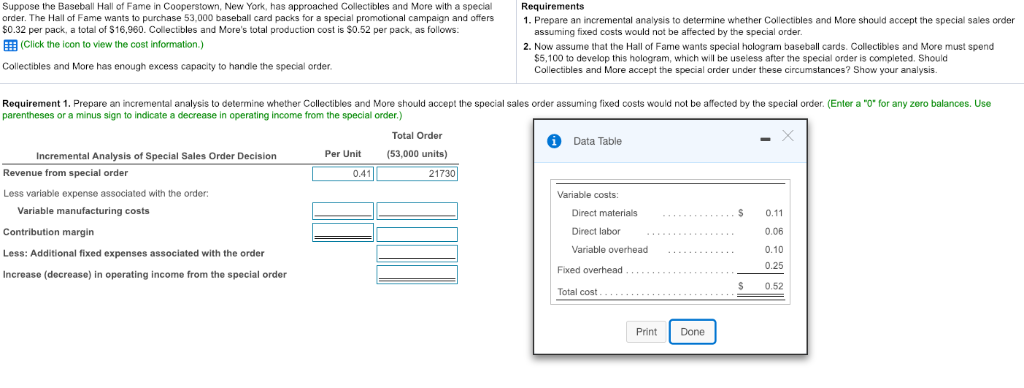Detailed Caption: 

The image depicts a detailed page from a financial analysis report. It begins with an introduction, stating that the Baseball Hall of Fame in Cooperstown, New York, has approached Collectibles and More with a special order. The Hall of Fame is interested in purchasing 53,000 baseball card packs for a promotional campaign, offering $0.32 per pack, totaling $16,960. This offer is juxtaposed with Collectibles and More's production cost of $0.52 per pack. 

The document guides the reader through preparing an incremental analysis to ascertain if Collectibles and More should accept the special order, assuming fixed costs remain unaffected. Instructions note to enter zero for any zero balances and to use parentheses or a minus sign for decreases in operating income. 

A chart labeled "Incremental Analysis of Special Sales Order Decision" appears, with columns for the per unit price and the total order price initially filled out, while other fields remain blank.

The second page continues with more detailed requirements, including a blue pop-up box titled "Data Table," listing variable costs: direct materials at $0.11, direct labor at $0.06, variable overhead at $0.10, and fixed overhead at $0.25, summing up to a total cost of $0.52 per pack. Below this data table are options to print or mark the task as done, with the "done" button highlighted in blue and the print button in gray.